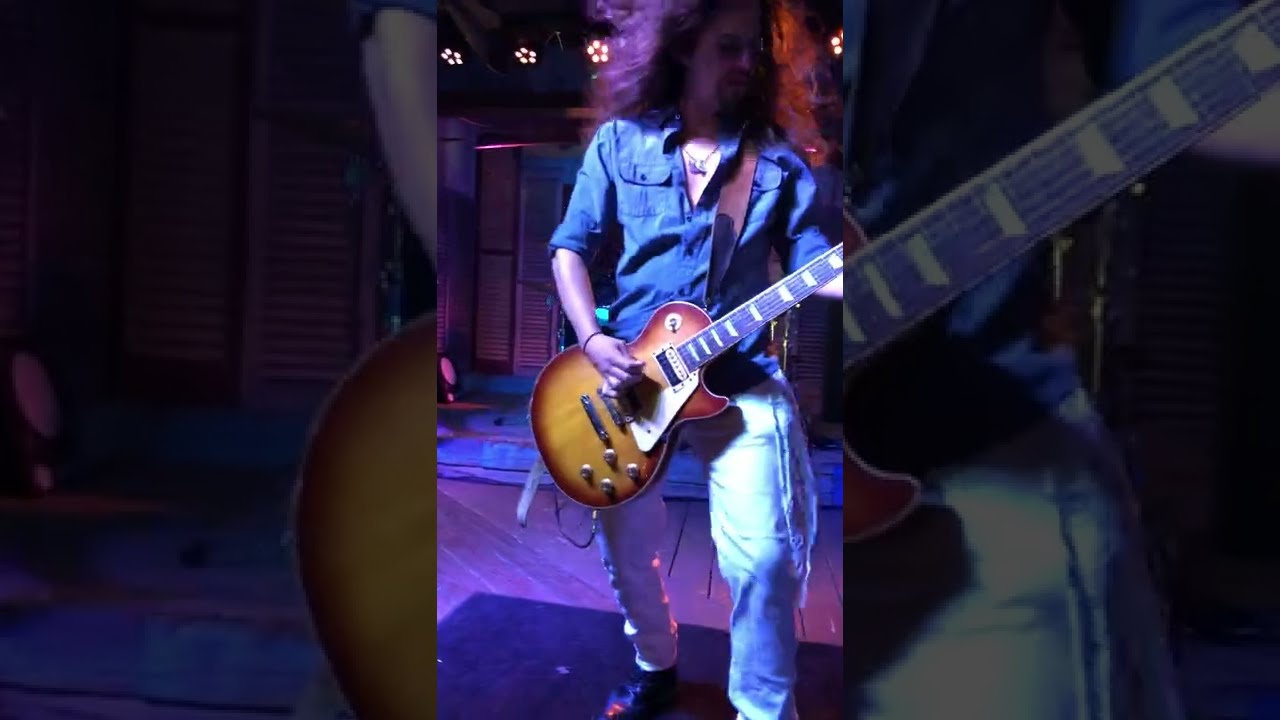In a dimly lit nightclub setting, a white male musician with long, dark brown hair combed back stands on a stage playing an electric bass guitar. He is dressed in a denim ensemble, featuring ripped blue jeans and an unbuttoned denim jacket which reveals a bare chest adorned with a necklace ending in a medallion. His right leg is pointed towards the audience while his left leg is positioned back, and he wears black shoes accented with orange tips.

His large, reflective sunglasses obscure his eyes, and his facial hair includes a goatee and mustache. He wears a wristband on his left arm. The guitar he cradles is predominantly brown with a burnt red or brick-colored edge and a section of white beside the strings. It includes four knobs and standard guitar strings. In the central shot, he is illuminated by stage lights above, while a close-up of the guitar's body occupies the left and right thirds of the image, merging into a spotlight on the musician at the center. His focused pose captures the intensity of his performance in the otherwise shadowed ambiance.